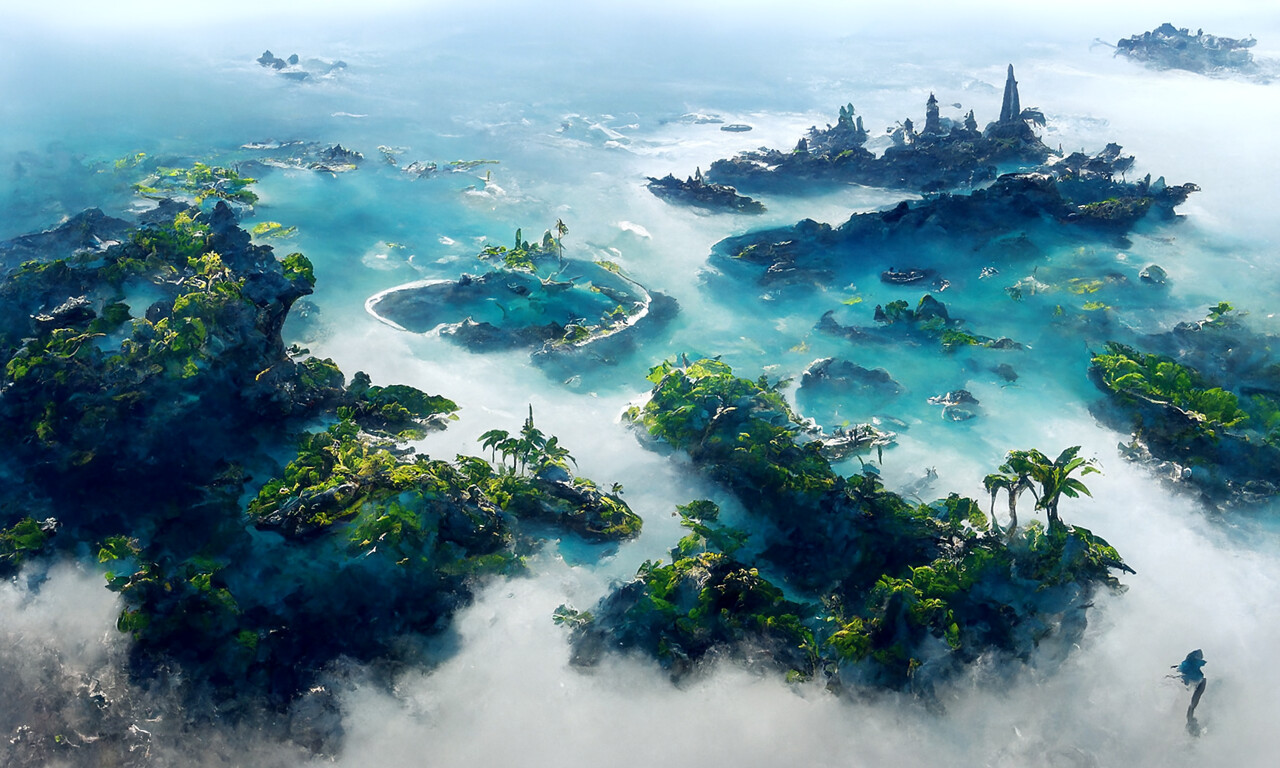This overhead image captures a fantastical, island-type environment with a vivid, video game-like style. Multiple scattered islands are set against a shiny, tropical blue ocean. The islands to the left feature lush, vibrant forests with hills, trees, and identifiable palm trees. Towards the top right, the landscape transitions into taller buildings and perhaps a small village nestled below a mountain. 

The central island forms a swirl pattern of rocky terrain punctuated by three patches of greenery. The bottom right island is predominantly rocky, with minimal plant life. Large rocks dominate these islands, with greenery covering parts but not all of them. In the background, a foggy or smoky area adds to the mystique, blending with the shiny blue water. The scene appears almost AI-generated with a detailed yet animated, fantastical quality, reminiscent of a movie set in a dreamlike world.